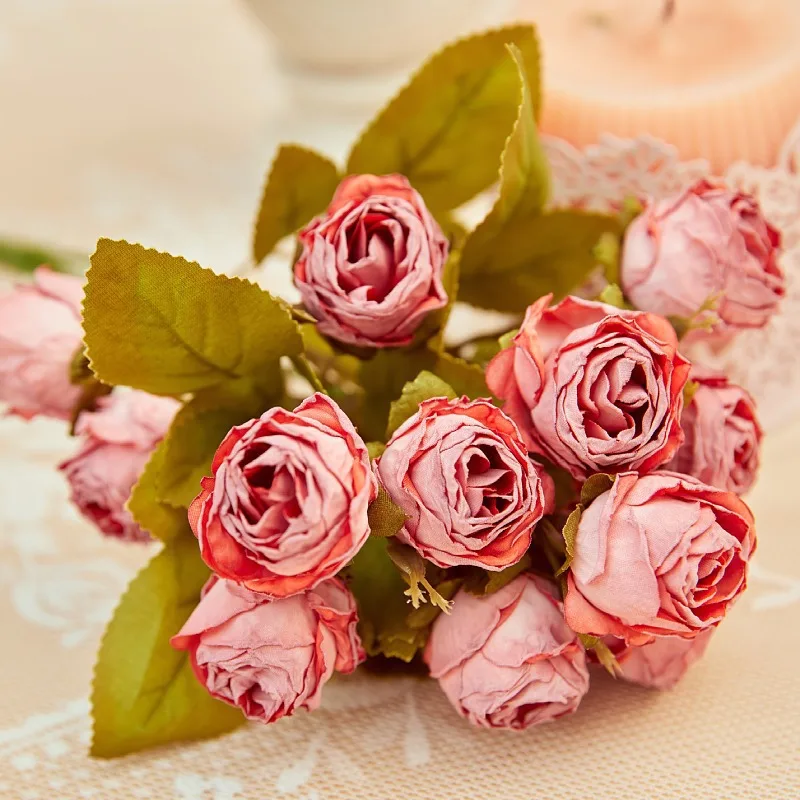This is a close-up photograph of a bouquet of around a dozen pink roses, lying on their side on a white and pink tablecloth. The image is taken from above, capturing the intricate details of the rose tops and their green leaves with a hint of yellow. The photograph is square in format and features a slightly blurred background, creating a shallow depth of field that highlights the flowers sharply while leaving some flowers in the background out of focus. In the upper right corner, there is a faint outline of a pink candle, and potentially a bowl behind it, adding to the still life composition. The surface beneath the roses has a light texture and the lighting is bright, suggesting that the photo was taken indoors.